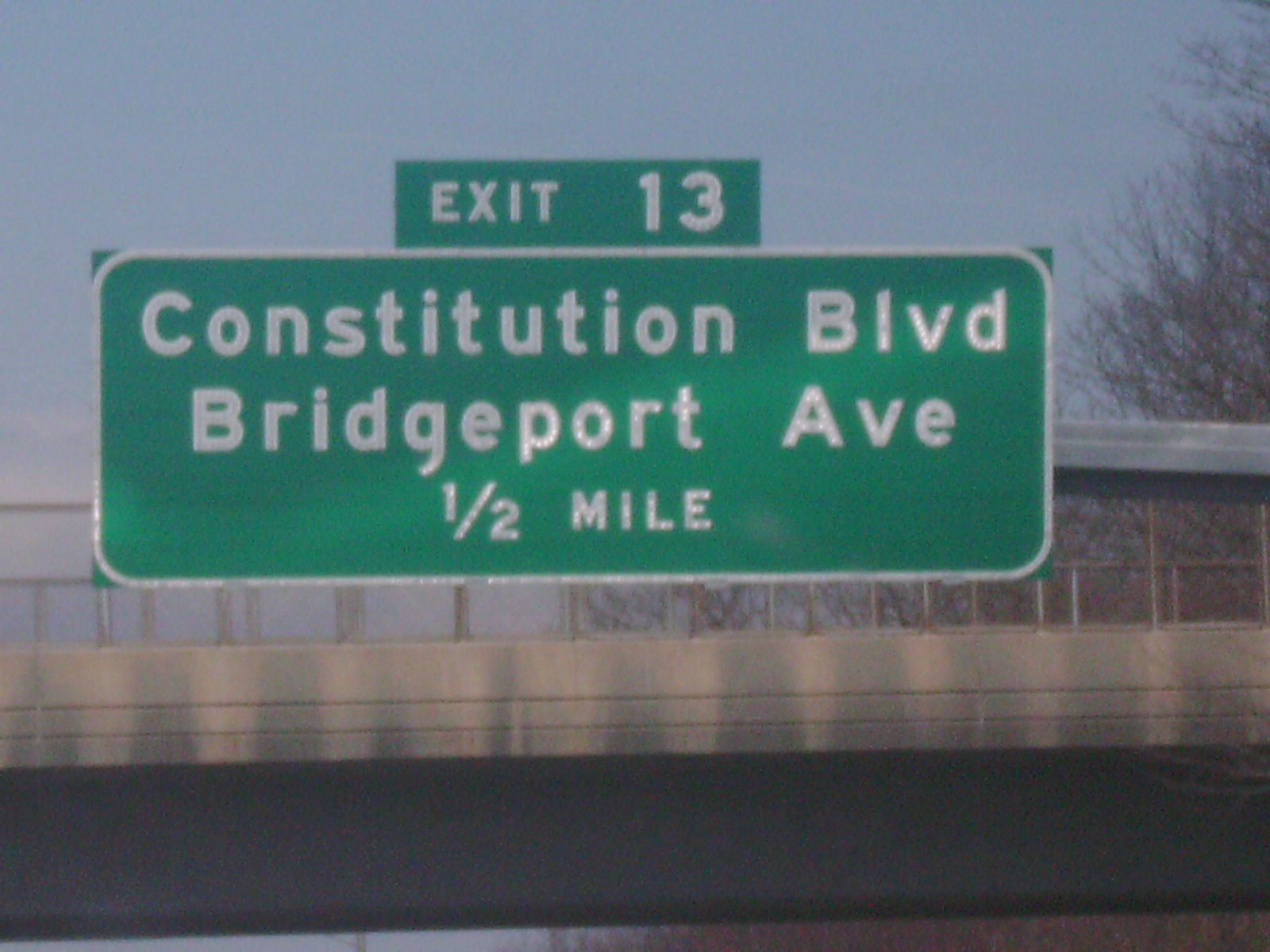A slightly out-of-focus photograph captures an overpass. At the bottom of the image, the underside of the overpass is visible, appearing dark with a cement structure directly above it. Prominently displayed above the cement portion is a large green highway sign bordered in white. The sign features white lettering that reads "Constitution B.L.V.D." followed by "Bridgeport Avenue A.V.E." beneath it. Additionally, it indicates "1/2 mile" as the distance. Above this is another green rectangular section with "EXIT 13" written in white letters. The background showcases a clear blue sky, and on the right side of the image, a tree devoid of leaves stands with its bare brown branches.